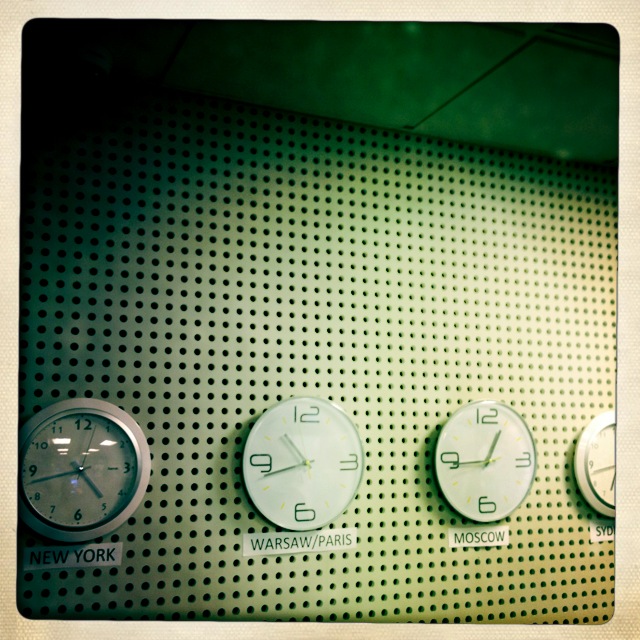A wall designed to resemble a perforated pegboard is adorned with four distinct clocks, each set to a different time zone. The first clock on the left is labeled "New York" and displays the time as approximately 4:43. This clock features a traditional design with numbers 1 through 12, a white rim, and a silver bezel encircling its glass face. The second clock, labeled "Warsaw/Paris," shows a time of around 10:43. Its minimalist face displays only the numbers 12, 3, 6, and 9, requiring interpretation for the other hours. The third clock, similar in design to the second, is marked "Moscow" and indicates a time close to 12:43. The final clock, partially cropped out of the image, bears the label "SYD," likely referring to Sydney, and seems to show a time of about 6:43. Each clock adds a unique touch to the wall, providing a snapshot of different times around the world.